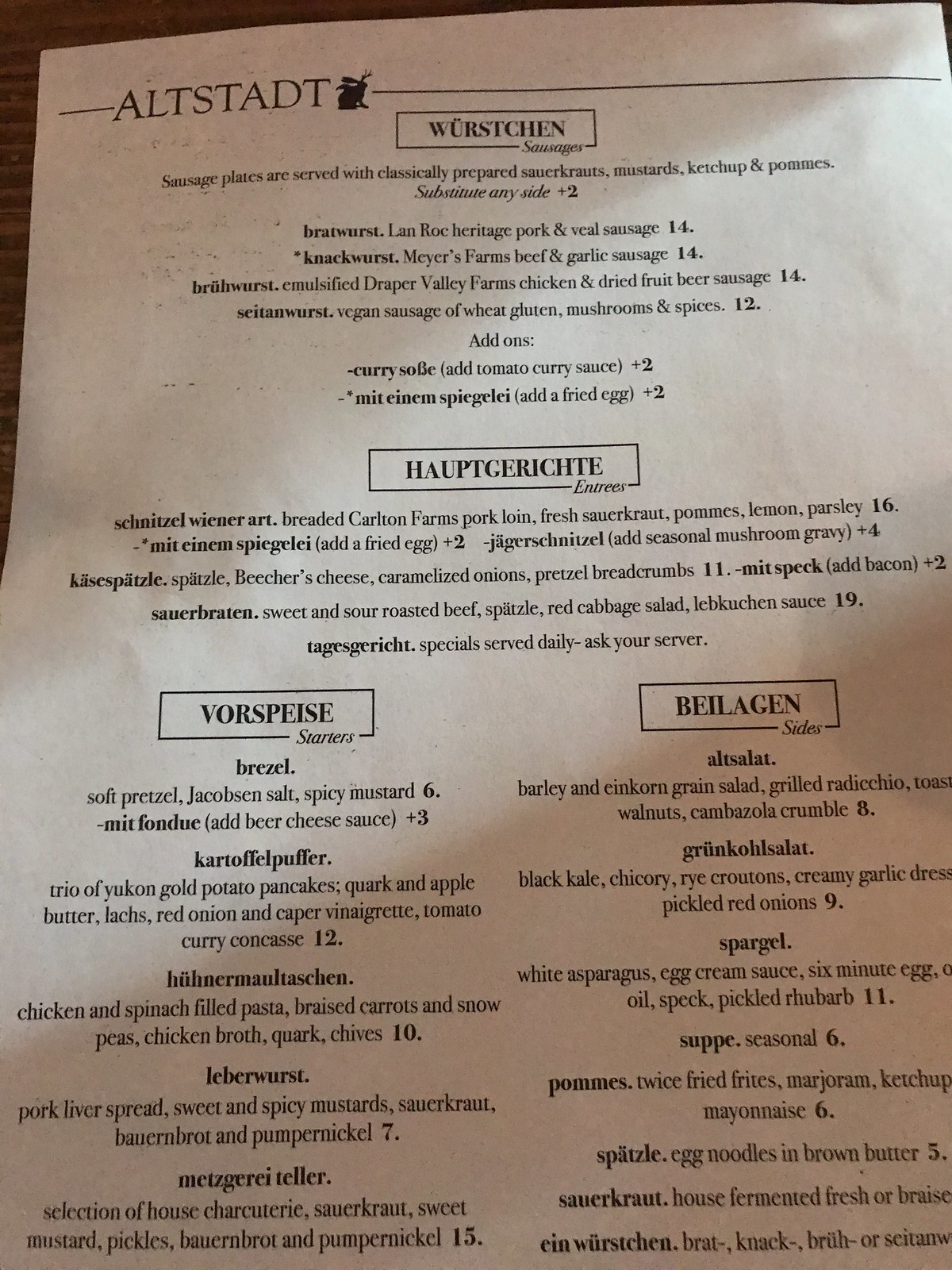The image features a menu mostly in a foreign language, set against a white background. A piece of brown wood is visible from the top left corner, angling down off the page about halfway, adding a rustic touch. 

At the top of the menu, a line emerges from the left side, leading to the text “Altstadt” with a small bunny rabbit outline beside it, giving it a quaint, charming feel. The line continues off the right side of the page. 

Centered on the menu is a black rectangular outline containing the word “Wurstchen” in black text. Below this heading are six food items listed, each detailing its contents from left to right and followed by their respective prices. 

Further down in the center, a black rectangle features the title “Hauptgerichte” (entrees), under which five items are listed. The composition of these dishes is described next to the item names, culminating with their prices on the right.

In the bottom half of the menu, there are two rectangular sections – one on the left and one on the right. 

The left rectangle is titled “Vorspeise” in bold letters with “starters” written underneath. It lists five starter items, detailing their ingredients below, and the prices listed to the right.

The right rectangle is labeled “Beilagen” with “sides” written just below it. Eight sides are listed here, with their ingredients detailed underneath and the prices listed beside them.